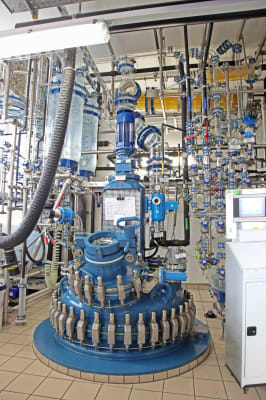The image depicts the interior of a cluttered science laboratory. Central to the scene is a large blue circular machine with a broad base which narrows towards the top. The base features numerous metal attachments resembling vertical silver knobs and interspersed zipper-like gray panels that encircle it. Surrounding this primary machine are several clear canisters and tubes, likely designed for fluid flow, although they currently appear dry. The machine sits atop a tiled floor that varies in description but seems predominantly light-colored. To the right of this central machine is a smaller, boxy white apparatus that might resemble a washing machine or cabinet. The background features additional machinery and tanks filled with fluid, and possibly glass shelves holding beakers and glass tubes of varying sizes. The room is illuminated by a ceiling light situated in the top-left part of the image, and a prominent pipe extends from the upper portion down to the left side of the photograph, adding to the industrial atmosphere of the space.